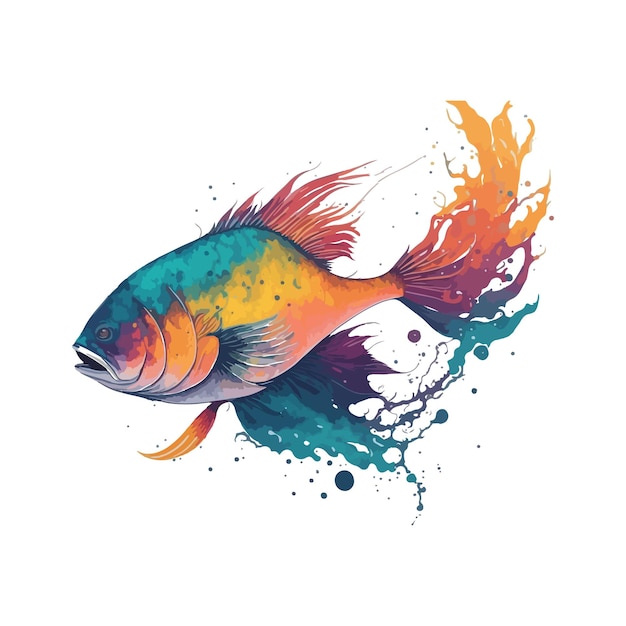The image is a vibrant and whimsical painting of a fish, depicted swimming to the left with its tail extending to the right. The fish's multicolored body features a harmonious blend of vivid hues, including aqua blue, teal, yellow, peachy orange, salmon, and various shades of purple. The head of the fish, covered in shades of green at the top, transitions into yellow and orange as it moves towards the middle. The gills, visible near the front, exhibit a gradient from purple to pink and then orange and yellow.

The fish's fins are artistically detailed and diverse in color. The top fin, resembling hair, is a mix of pink and reddish-orange, while the bottom fin has shades of blue, dark blue, and purple, with an additional smaller fin colored in yellow, red, and purple. The back fin combines yellow, orange, purple, and blue, artistically dissolving into wispy trails and droplets of paint, giving the impression of motion and creation. This effect is mirrored in the tail fin, which extends out in shades of orange, purple, and teal, appearing as though it is gently disintegrating into colorful dots.

The fish's slightly open mouth is outlined in white, emphasizing its whimsical appearance. Surrounding the fish are multicolored bubbles and circles, primarily in blue and purple. The background of the painting is stark white, which enhances the vivid colors and artistic detailing of the fish, making it appear as though it is floating in an ethereal, otherworldly environment. The overall effect of the painting suggests a fanciful and imaginative representation, reminiscent of styles found in digital art or watercolor mediums.